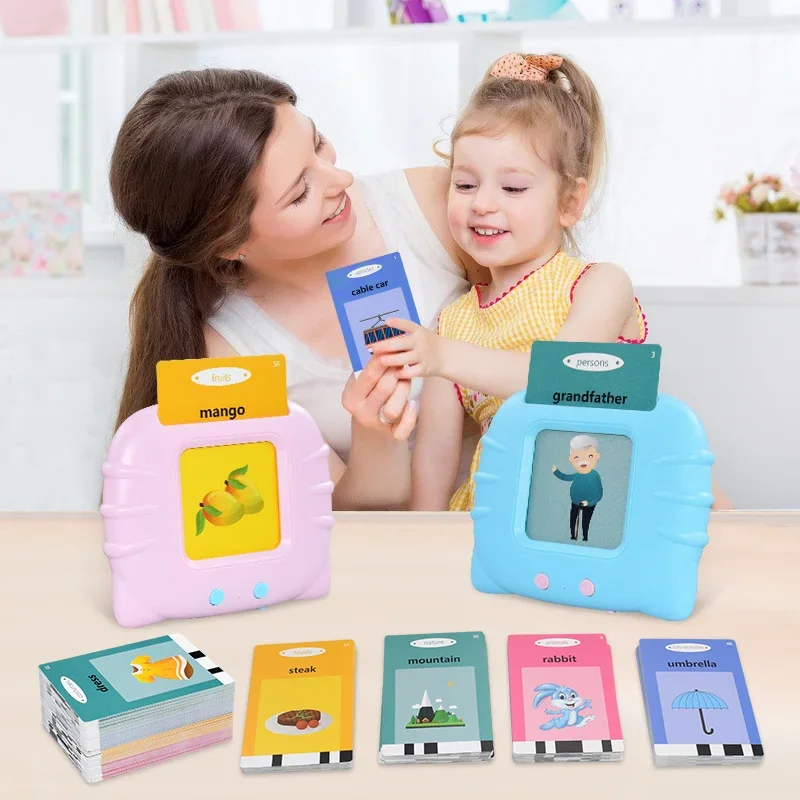The photo captures a touching scene of a mother and her little girl, likely in a bright and cheerful nursery setting. Both are engaged in an educational activity using a set of colorful flash cards. The mother lovingly holds her daughter on her lap as they explore the cards together. In front of them, there are two plastic devices resembling picture frames, each equipped with two buttons – one pink with blue buttons and the other blue with pink buttons – designed to hold the flash cards.

The table in front of them is tan and holds a substantial deck of cards off to the left, organized by various categories such as food, nature, animals, and fruits. Visible cards include a blue one with an umbrella, a pink one with a rabbit, a green one with a mountain, and a yellow one featuring a steak. The mother and daughter are both holding a blue card labeled "cable car," while other cards displayed in the devices show a "grandfather" card and a "fruits mango" card. The background is bright, enhancing the joyful and educational atmosphere of the scene.